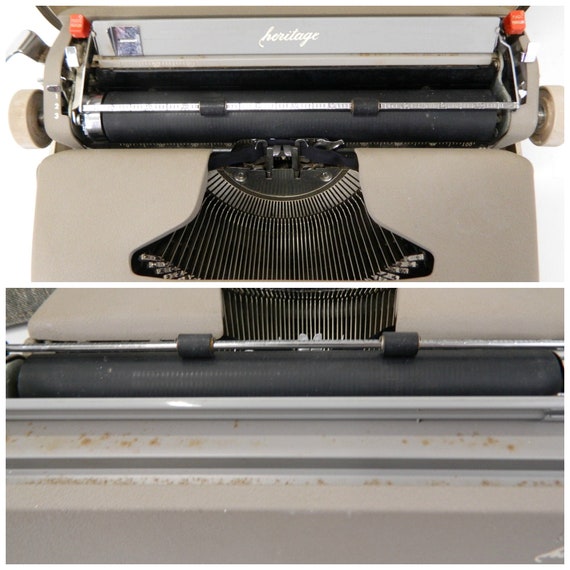The image comprises two photographs of a vintage Heritage typewriter, prominently displaying the brand name "Heritage" in white script across the top. The typewriter, a blend of gray, black, and potentially silver from its metallic components, dominates both shots with no other items in view. In the top half, we see a bird's-eye view of the typewriter with its keyboard removed, revealing the exposed metal keys and a round ink roll at the center. The bottom half presents a reversed bird's-eye perspective, showcasing the same typewriter but from an opposite angle, emphasizing the machine's intricate metal workings. The overall composition highlights the mechanical elegance and timeless design of this retro device, rich in detail from the circular paper knobs on top to the slightly rusted arms of the typewriter mechanism.